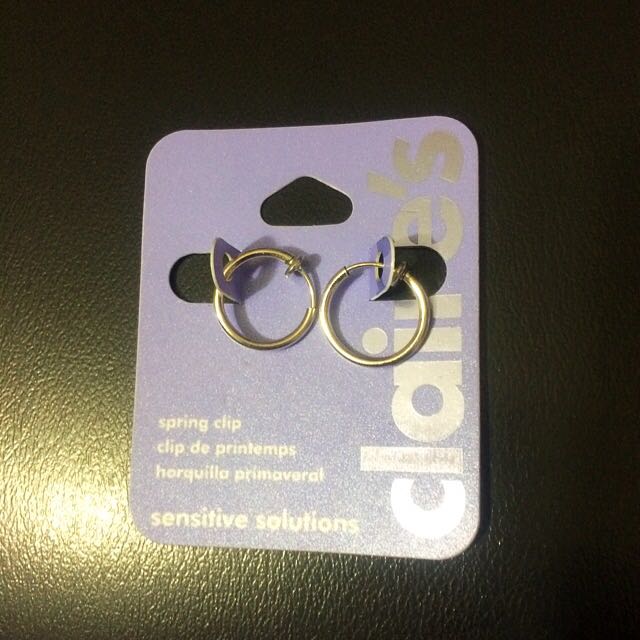This image features a brand new pair of circular gold hoop earrings presented on a purple cardboard display card, likely purchased recently from Claire's. The card, which has cutouts for hanging and attaching the earrings, prominently displays the brand name 'Claire's' in vertical white lettering on the right side. On the bottom left of the card, the text reads "Spring Clip," "Clip de Printemps," "Horkula Promethea," and "Sensitive Solutions," all in a smaller white or gold font. The black background, possibly leather or faux leather, creates a striking contrast, with a light source illuminating the lower left-hand corner. The overall image is detailed but not perfectly focused, emphasizing the luxurious appeal of the earrings.